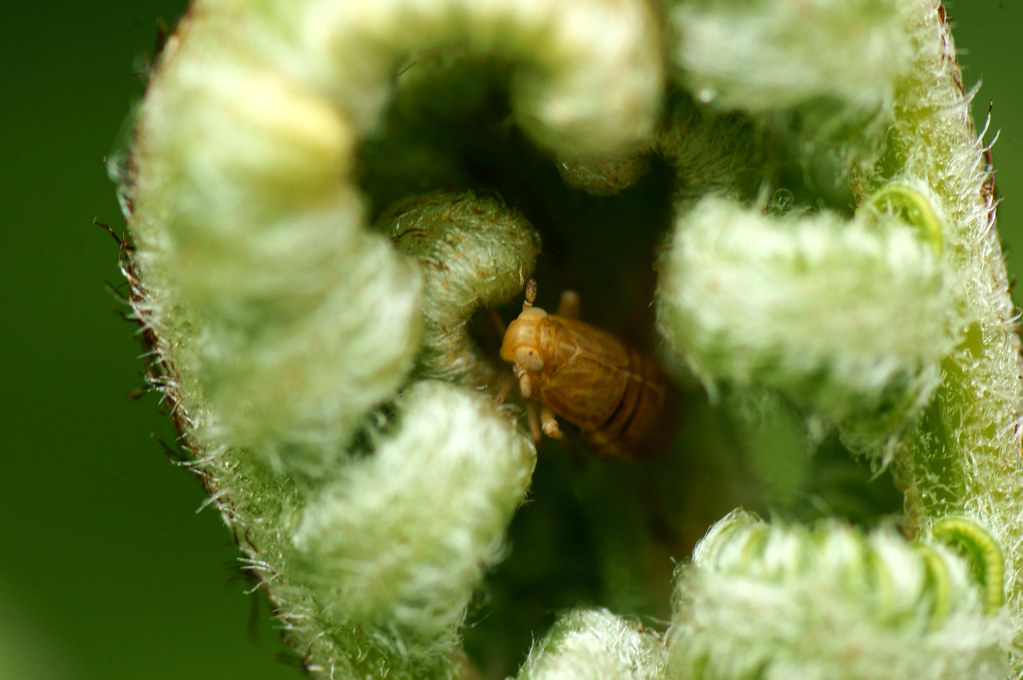In this vivid close-up image, we see an intriguing plant or organism, possibly resembling a cacti or a green flower, with an open, hand-like structure curling around a central cavity. Within this cavity rests a yellowish-tan insect, perhaps a young grasshopper or cicada, characterized by its puffy eyes and stubby arms. The insect's detailed features, combined with the light green and brown hues of the plant, create a striking contrast. The hazy, light green background enhances the focus on the plant and insect, while the ambient sunlight gently illuminates the scene, emphasizing the lush green of the foreground and adding depth to the overall image.